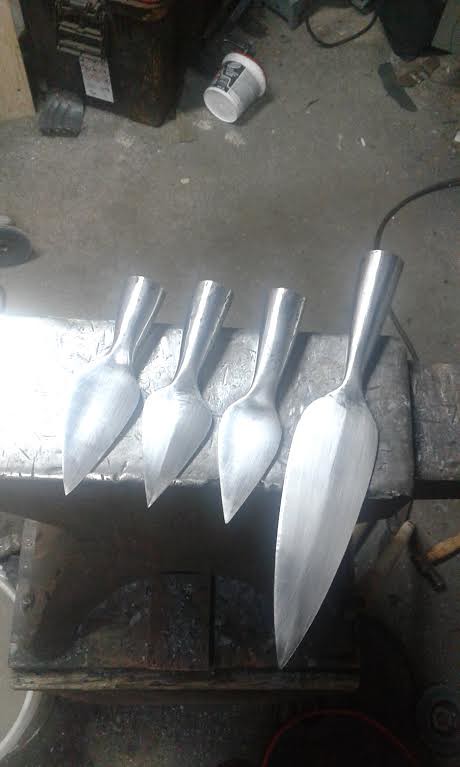This close-up color photograph showcases four silver utensils, possibly gardening tools or specialized knives, carefully balanced on an aged, black metallic surface that is likely part of an old grill. Each utensil has a spherical end with a rounded handle, and they vary in size. The one on the far right is significantly longer, with both a longer handle and blade, while the other three are short and similar in size. This setup is situated in a dingy, workshop-like setting, evidenced by the concrete floor that appears dirty and worn. In the background, a white plastic container lies on its side next to a rusted, black machine, which could be a battery charger. The space seems cluttered, with black storage bins partially visible in the top-left corner. This detailed scene evokes a sense of abandonment and utilitarian use, highlighted by the contrasted lighting on the metallic surfaces.